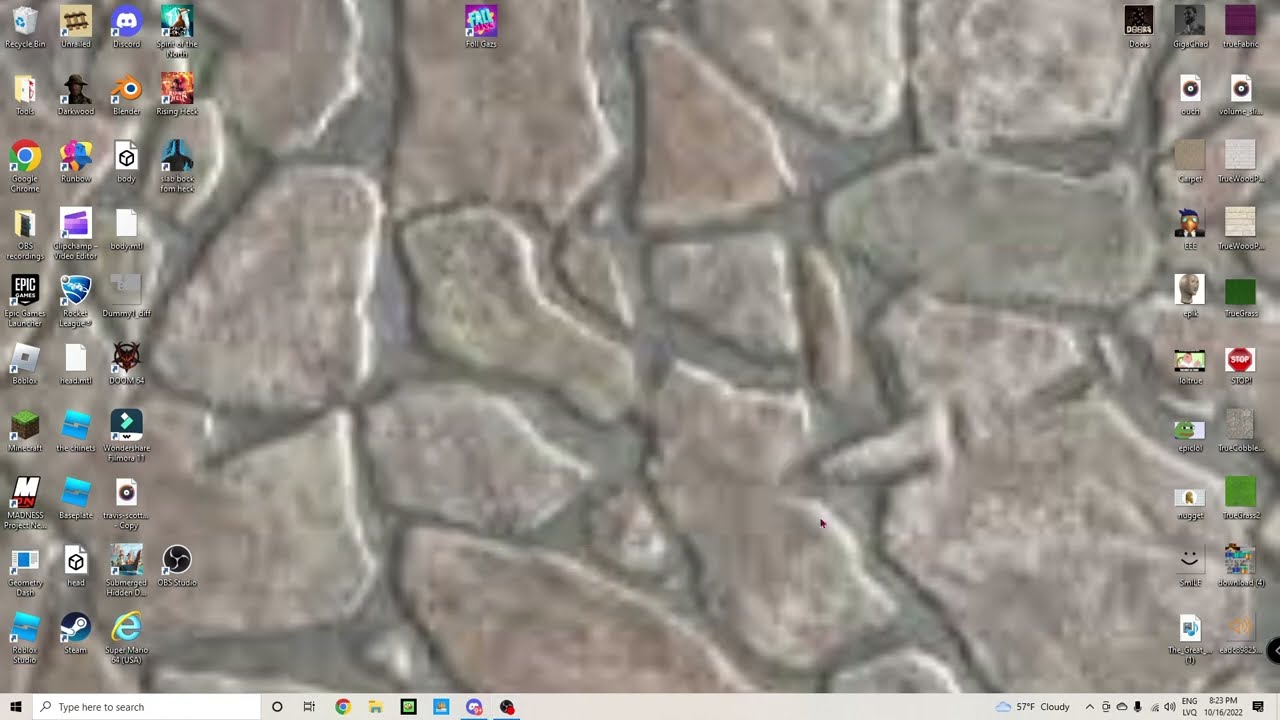This image is a screen capture of a Windows desktop. The background wallpaper features an overhead shot of patio stones, exhibiting a blend of gray and pinkish hues separated by gray mortar, though the image appears blurry and pixelated. The desktop is highly organized, populated with numerous icons aligned in rows on both the left and right sides of the screen. Notable icons include Minecraft, Recycle Bin, Discord, Blender, Google Chrome, Internet Explorer, and Steam, indicating a variety of software and applications. In the top center, there is a folder or file named "Fell G A Z S," possibly referring to the game "Fall Guys." The gray taskbar at the bottom of the screen includes a black Windows icon on the left, followed by a light gray search bar and various colorful program icons (green, blue, purple, black). On the right side of the taskbar, the time, date, Wi-Fi signal, and temperature (noting it is cloudy) are displayed, providing a full view of the user's desktop arrangement.